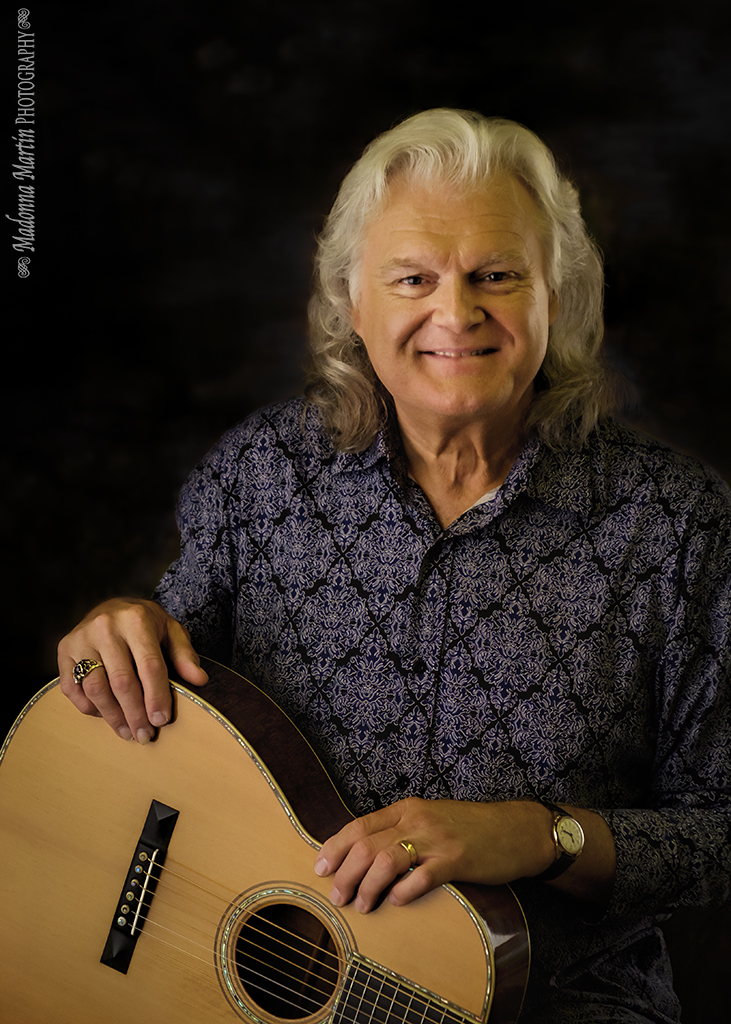In the professionally shot studio photo by Madonna Martin Photography, an older man, seemingly in his 60s or 70s, poses and smiles warmly for the camera. He has long, shoulder-length white hair, slightly balding in the front, and is clearly of Caucasian descent. The man is dressed in a blue button-up shirt adorned with a white paisley and diamond floral pattern. On his left wrist, he sports a watch, and he wears rings on both hands. The acoustic guitar he holds is distinctive with a yellow body and brown sides, and he grasps it in an unusual manner, with the neck facing down and positioned to the left. The entire scene is set against a pitch-black background, which accentuates the subject and his instrument. The upper left corner of the image features a watermark crediting "Madonna Martin Photography" in white text.